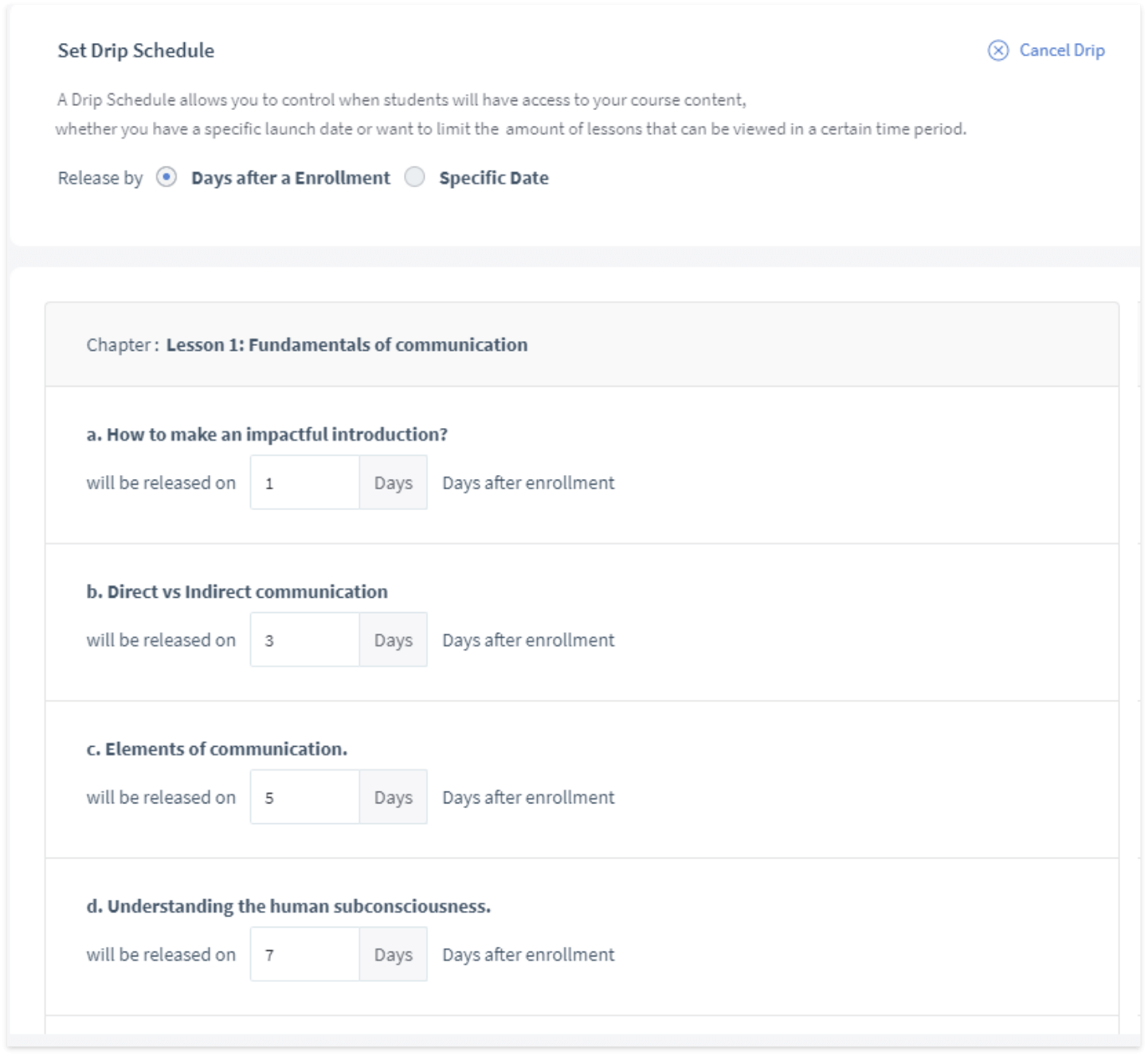A screenshot of a course management interface titled "Set Drip Schedule" is displayed prominently at the top in black text. The interface explains that a drip schedule allows instructors to control when students access course content, whether it’s through a specific launch date or by limiting the number of lessons available over a certain time period. 

Two options are available for releasing content: "days after enrollment" or on a "specific date." 

Below this, the course’s content schedule is outlined in detail:

- **Chapter: Lesson 1, Fundamentals of Communication** (in bold text)
  - **A. How to Make an Impactful Introduction**: This lesson will be available 1 day after enrollment. The "1 day" is editable.
  - **B. Direct vs. Indirect Communication**: This lesson will be released 3 days after enrollment. The "3 days" is editable.
  - **C. Elements of Communication**: This lesson will go live 5 days after enrollment. The "5 days" is editable.
  - **D. Understanding the Human Subconsciousness**: This lesson will be accessible 7 days after enrollment. The "7 days" is editable.

All headers (A, B, C, D) are in bold text, with descriptions beneath them in plain black text. This setup seems to be part of an editable teacher course platform that ensures the incremental release of curriculum to students.